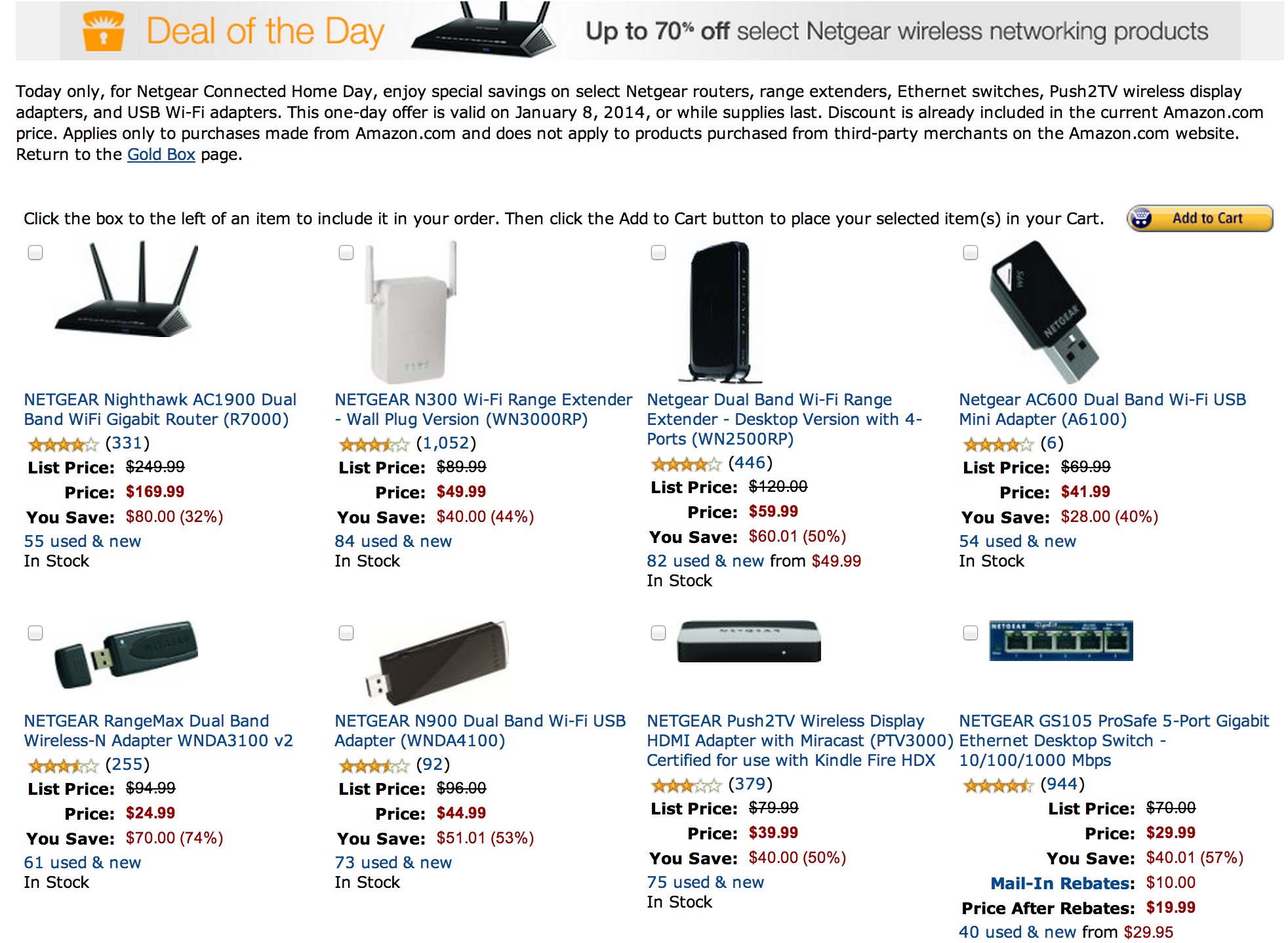This image captures the 'Deal of the Day,' highlighting a selection of Netgear products available at significant discounts. At the top, a gray rectangular banner features an orange text reading 'Deal of the Day,' accompanied by an orange logo resembling an opening box on its left. Central to the image is a prominent picture of a black Netgear router. To its right, bold text announces discounts of up to 70% on select Netgear wireless networking products.

Beneath this main section, there are eight smaller product images arranged in two rows. The top row showcases:

1. A black Netgear Nighthawk router.
2. A white Netgear Wi-Fi range extender.
3. A black Netgear dual band Wi-Fi range extender.
4. A Netgear dual band Wi-Fi USB adapter.

The bottom row includes:

5. A black Netgear RangeMax dual band adapter.
6. A black Netgear Wi-Fi USB adapter.
7. A black and gray Netgear wireless display HDMI adapter.
8. A Netgear 5-port gigabyte ethernet desktop switch.

Each product image is followed by a description in blue text, a star rating, a crossed-out list price, the current discounted price, and the total savings.